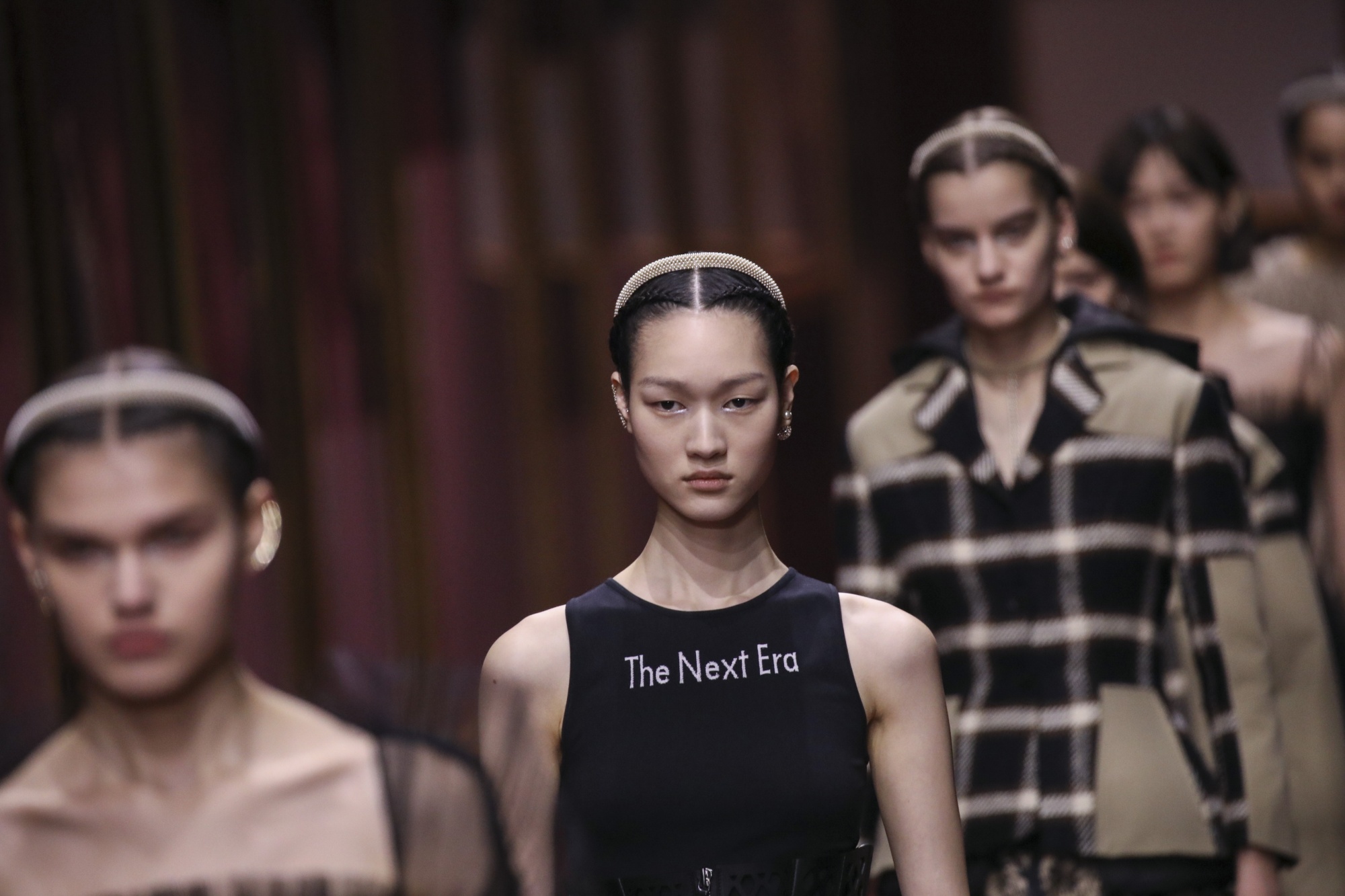The image captures an indoor fashion runway show featuring a line of female models with their hair slicked back and styled into tight braids that form a heart-like shape at the front, all adorned with white headbands. The central focus is on a strikingly beautiful model of Asian descent, wearing a black sleeveless halter top emblazoned with the words "The Next Era" in white lettering. She exudes fierceness as she gazes ahead, her long, thin neck accentuated by gold dangly earrings and a natural, makeup-free look. The background is blurred, revealing indistinct figures of other models dressed in a variety of outfits, enhancing the sense of movement and diversity typical of a dynamic fashion show. In the far background, there appears to be reddish-brown curtains, adding a touch of warmth to the setting.